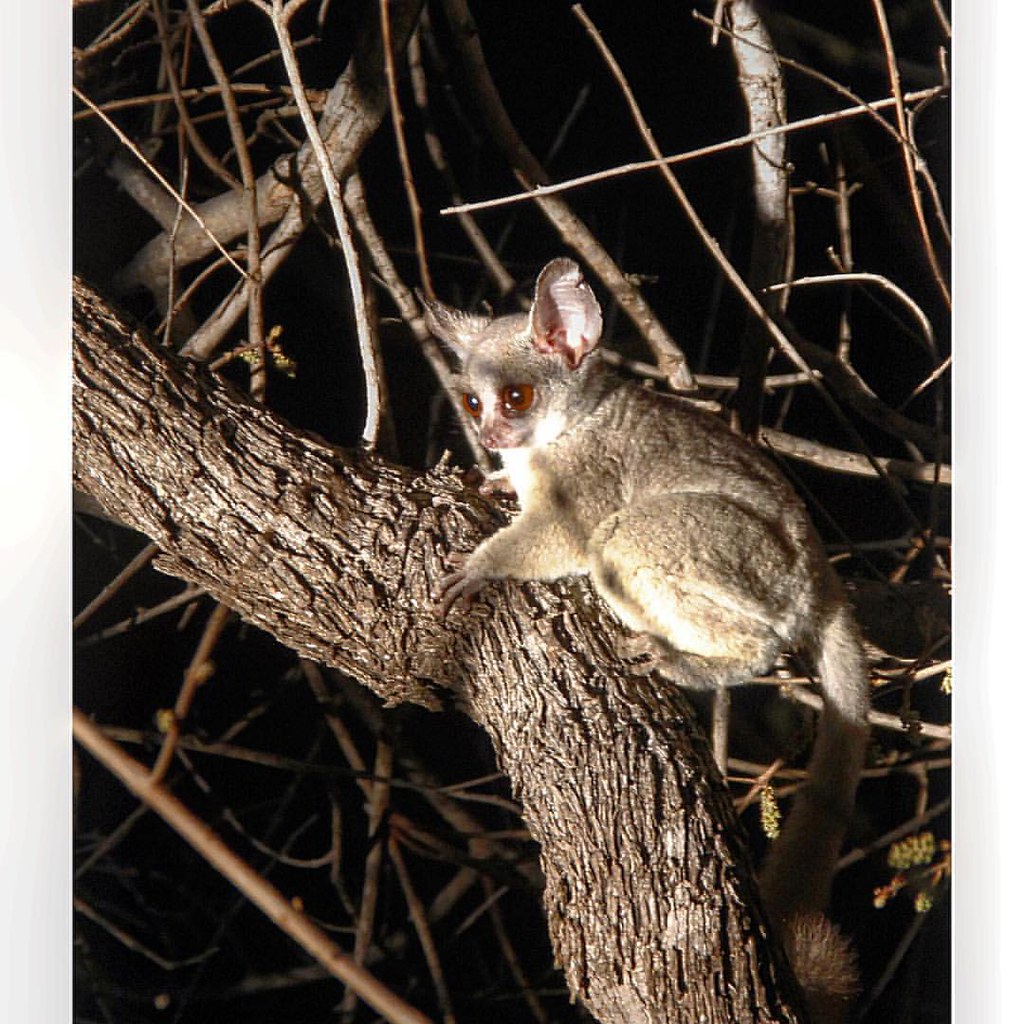The image depicts a nighttime scene illuminated by a light source, which reveals the intricate details of a tree with numerous branches that extend throughout the frame. At the center of the image, perched on one of the sturdier branches, stands a small, grayish-white mammal, likely a monkey, identifiable by its distinctive bat-like features, including large, upright ears and big, orange-brown eyes. The monkey's side profile shows it gazing off to the left, showcasing its sharp front claws and a long tail that begins white and transitions to a brownish hue towards the end. Scattered among the branches are some leaves or berries, adding subtle splashes of green to the predominantly dark and muted color palette composed of blacks, grays, and browns. The scene appears to be set outdoors at night, possibly on someone's property, with a pitch-black sky serving as the backdrop.